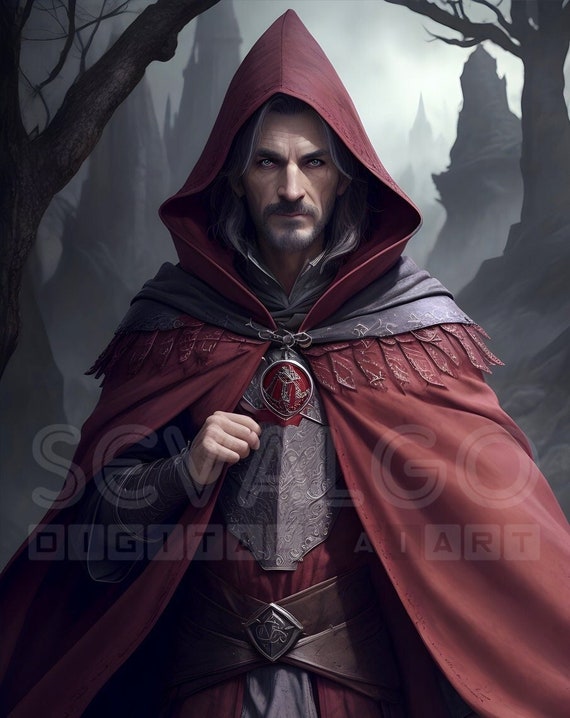This AI-generated digital artwork, marked as "Sovalgo digital AI art," depicts a wizard-like man with long, gray hair and a gray goatee. He has light gray, glowing eyes set against pale skin, and is dressed in a pointed hooded red cloak with a gray shawl draped over it. The cloak, detailed with smooth, metal decorations and red and gray tones, is complemented by a maroon outfit and metal armor underneath, including a metal waistband. The wizard's right hand is raised to his chest, while his left hand remains hidden under the cloak. A prominent red amulet is visible at his neck. The background features a foggy and eerie landscape with leafless trees, large castles, rocky terrain, and distant hilly areas, all contributing to a dark and mystical atmosphere.